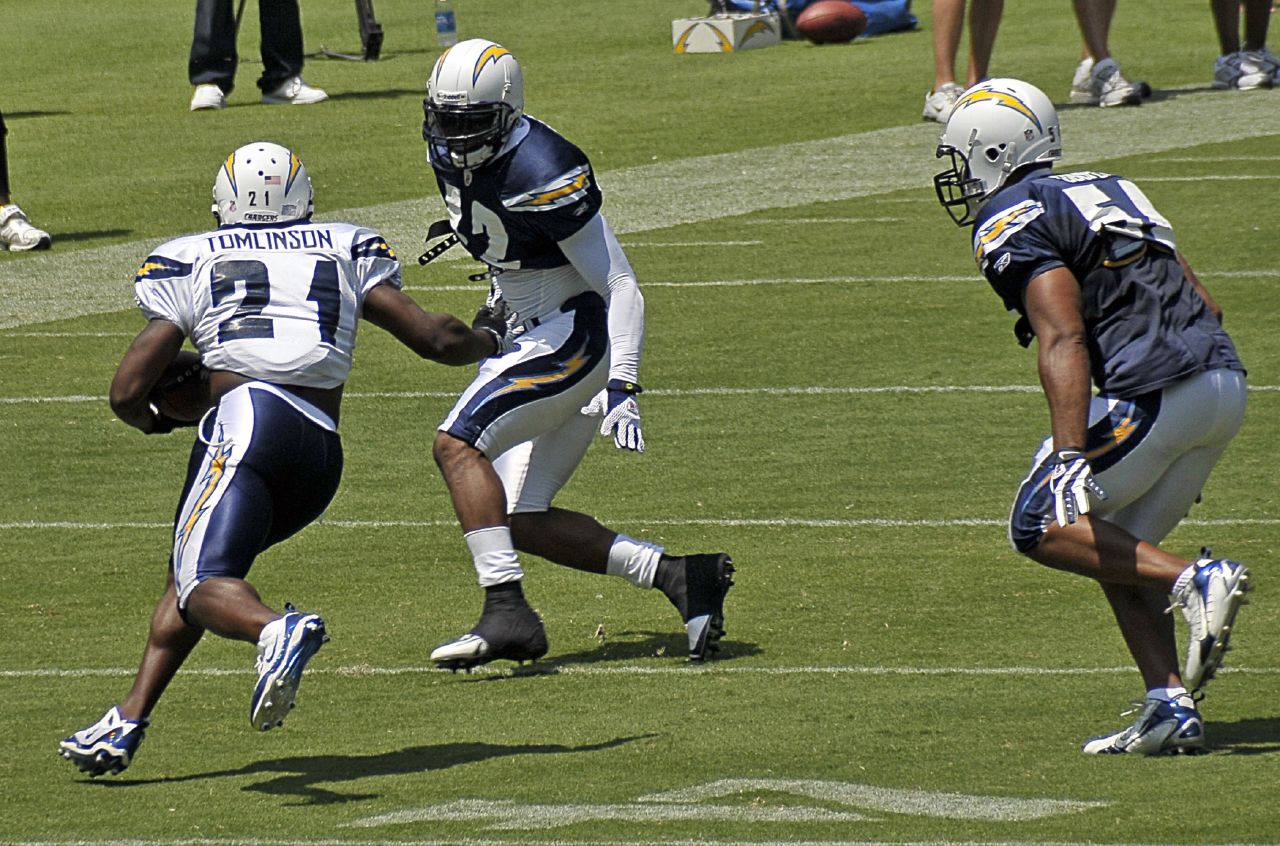In this detailed image, we see a practice session for the Los Angeles Chargers football team taking place on a football field. At the center of the action is LaDainian Tomlinson, wearing a white jersey with the number 21 and his name above it, prominently displayed in black. His helmet features two distinctive yellow lightning bolts. Tomlinson is carrying the football and appears to be trying to evade two defensive players. The defenders are clad in dark blue jerseys and white pants, contrasting with Tomlinson's lighter attire. Both defenders wear black shoes, while Tomlinson is in white footwear. The composition places one player towards the right middle and the other two towards the left middle of the frame. The defensive player on the left is positioned towards the bottom left corner, adding dynamism to the scene.

In the background, we can make out the legs of the trainers and coaches stationed along the edges of the field, hinting at their observant presence without detracting from the main action. Scattered footballs, team logos, and practice equipment can be seen across the expanse of the turf field that stretches into the distance. The absence of bleachers reinforces the setting as a practice field. The color palette is dominated by dark blue, white, yellow, light brown (for the football), brown, tan, and black, adding to the authenticity and vibrancy of this practice scenario.